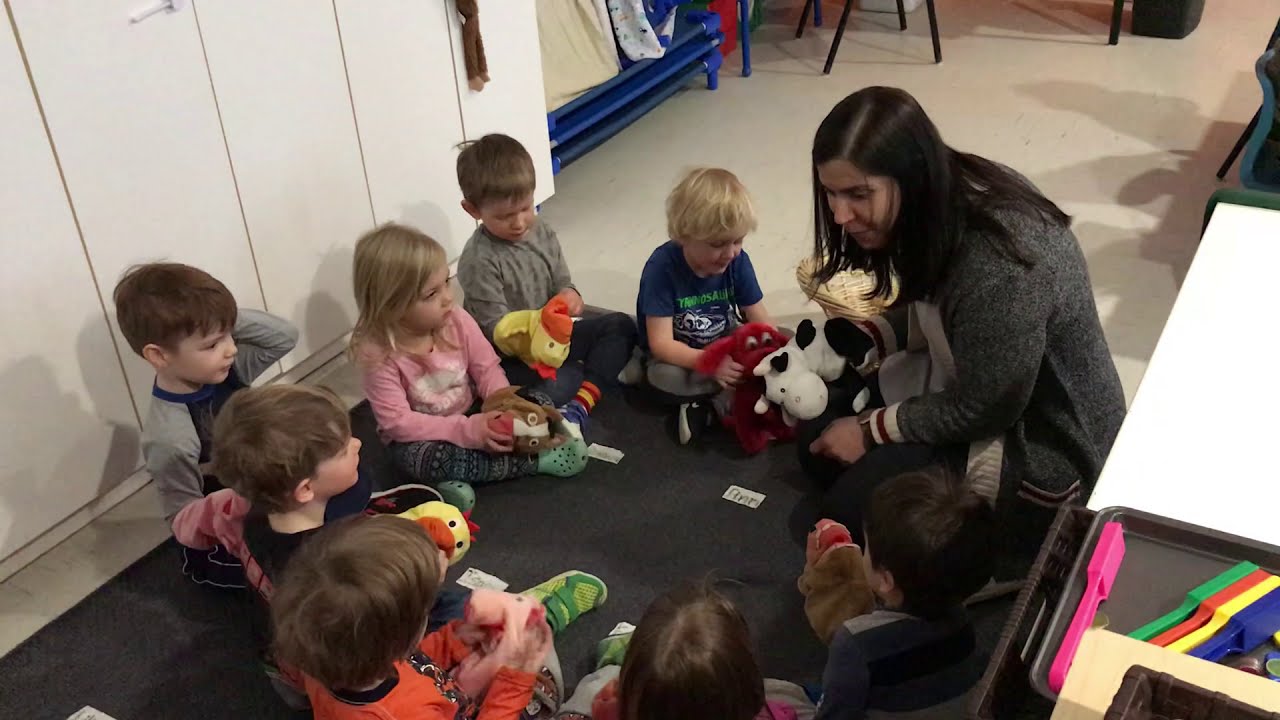In this indoor preschool classroom, a group of eight children, approximately four years old, are seated in a circle around an adult, likely their teacher, who is wearing a gray hoodie. The children and the teacher are engaged in an activity involving stuffed animals, which include a yellow and orange duck, a red dog, a black and white cow, a pink pig, a green dinosaur, and other colorful and whimsical creatures. The child next to the teacher has blonde hair and is wearing a blue shirt, while other children are dressed in variously colored outfits, including gray and dark pants, pink and patterned pants, and an orange shirt. They are sitting on a gray mat in front of a backdrop of white cabinets or lockers. Towards the back of the room, the feet of black chairs and a white table are visible, along with a blue coat rack with garments hanging. In the lower-right corner of the image, there is a tray with colorful, plastic instruments that are likely magnets, in pink, green, orange, yellow, and blue. The scene depicts a lively and engaging educational environment.